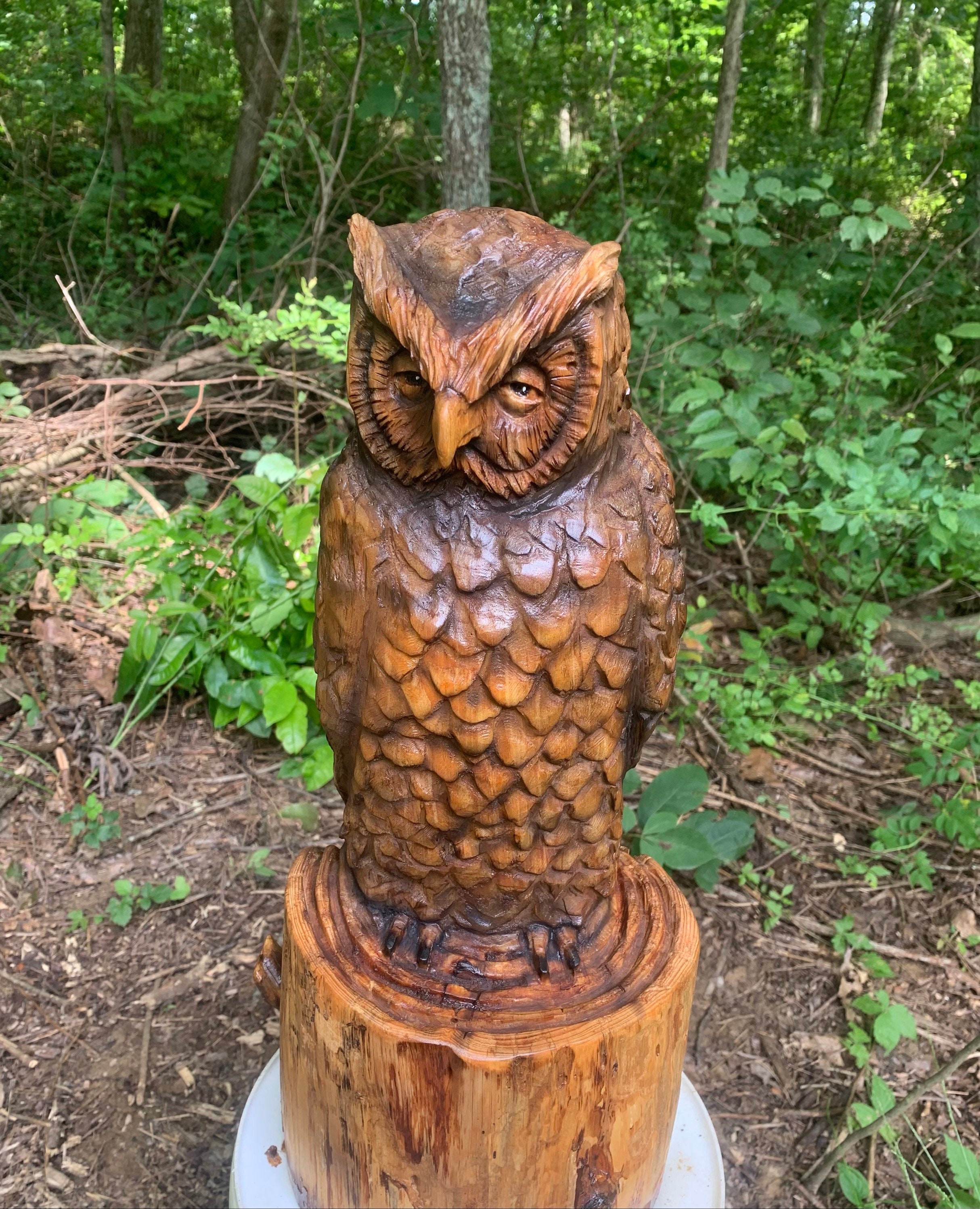In this detailed image, a meticulously handcrafted wooden owl sculpture stands prominently in a woodland setting. The owl, featuring intricately carved facial features, detailed feather layers, and visible individual claws, is perched on top of a log that rests on a white platform. This platform sits directly on a forest floor, scattered with dirt, brown leaves, and fallen sticks. The scene is captured during the day, with sunlight filtering through the trees. In the background, a natural opening in the woods reveals a variety of foliage, including bushes, branches, and additional broken wood, enhancing the rustic, forest ambiance of the photograph. No text or other objects disrupt the focus on the owl and its natural surroundings.